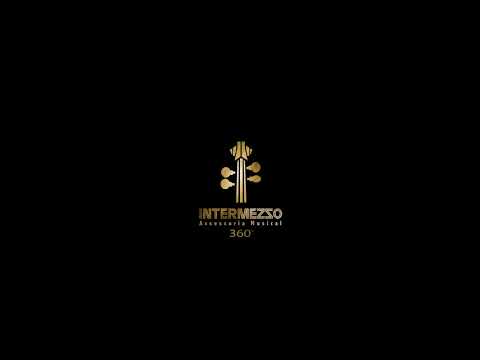The image is a graphic representation designed for a likely PowerPoint slide, centered around a business logo. The entire frame is solid black, emphasizing the central logo, which resembles the headstock of a stringed instrument like a guitar or possibly a cello, featuring four tuning pegs on either side. The logo, in a pale gold to white gradient, displays the word "Intermezzo" in bold print, with the second "Z" reversed. Below "Intermezzo," there are two smaller, unreadable words, followed by the number "360," hinting at possible services related to 360 photography or virtual reality themes. The overall design is simple yet striking, with the logo and text standing out sharply against the dark background.